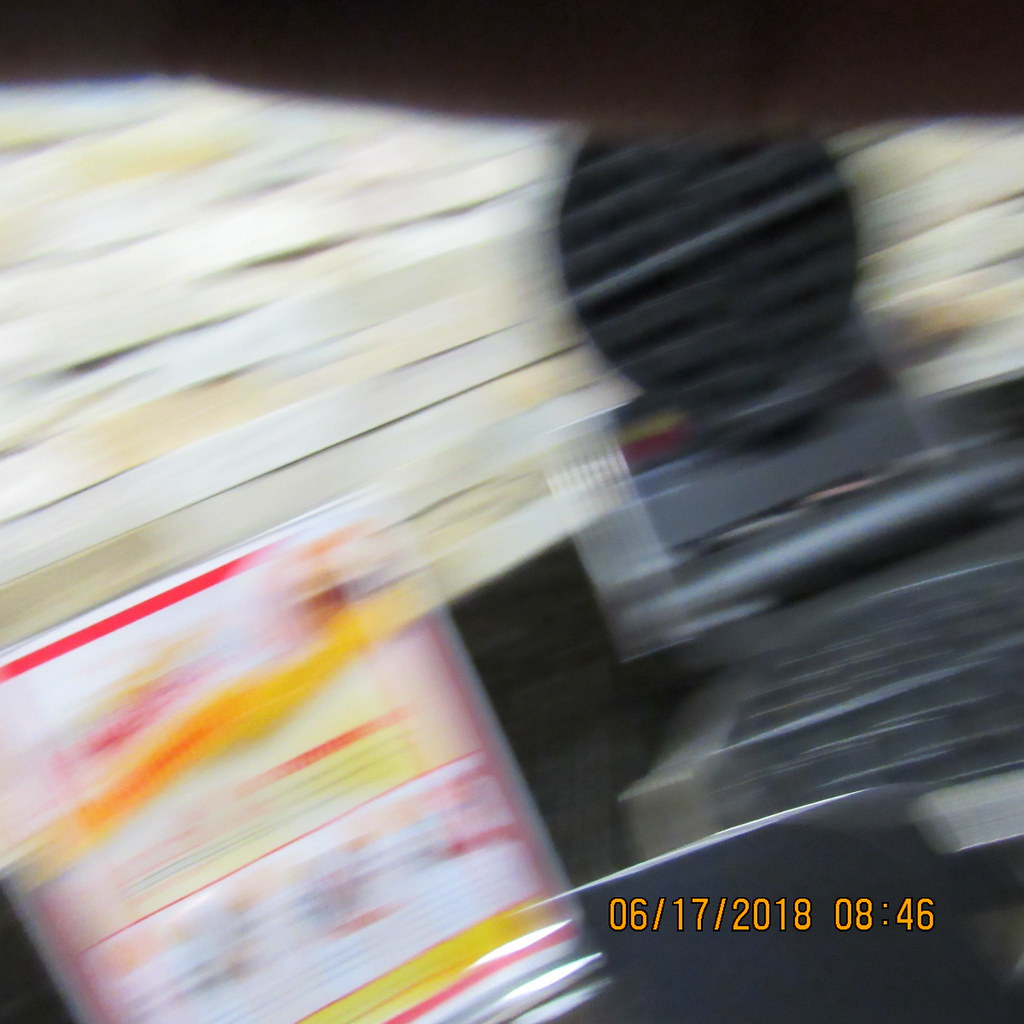The image depicts a highly blurred scene caused by the camera being moved rapidly from the bottom left corner to the top right corner. In the bottom right corner of the photo, an orange date stamp reads "06-17-2018 at 08-46". Amidst the blur, a white box is discernible on the left side, reminiscent of a cake mix box. This box is bordered by a red line and appears to have directions or instructions printed on it, with a noticeable yellow section on the back. Adjacent to this box is a gray object, possibly a cash register, with a prominent dark circular feature perched atop it. The motion blur makes it challenging to ascertain finer details, but the general shapes and colors are still partially identifiable.